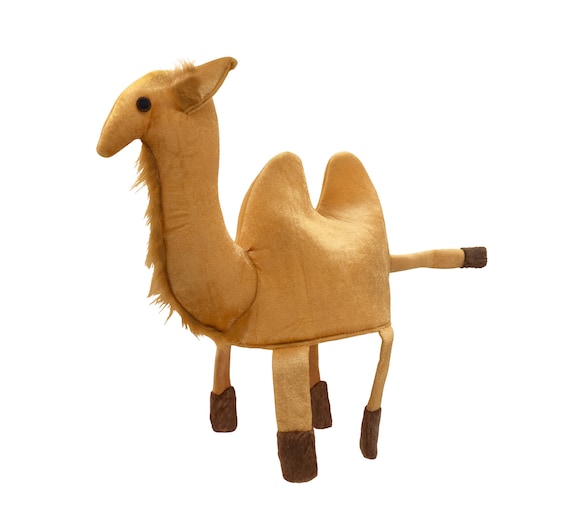In this photograph set against a crisp white background, we see a small stuffed toy camel. Tan in color, the camel is depicted in profile, facing left. It has two distinct humps on its back, characteristic of its species, and its beady black eyes and upward-pointing ears are clearly visible. The camel’s body is plush, likely filled with cotton, giving it a soft and slightly floppy appearance. Its four legs, crafted from the same tan fabric as the body, end in dark brown rectangular feet, adding to its charmingly simple design. There’s a strip of felt "hair" running down its long neck and small tufts in its ears. Completing the figure is a tan tail with a dark brown pad at its end, mirroring the legs. This lovingly made toy, possibly a local artisan’s craft, brings a sense of whimsy and authenticity, making it a delightful souvenir for tourists.